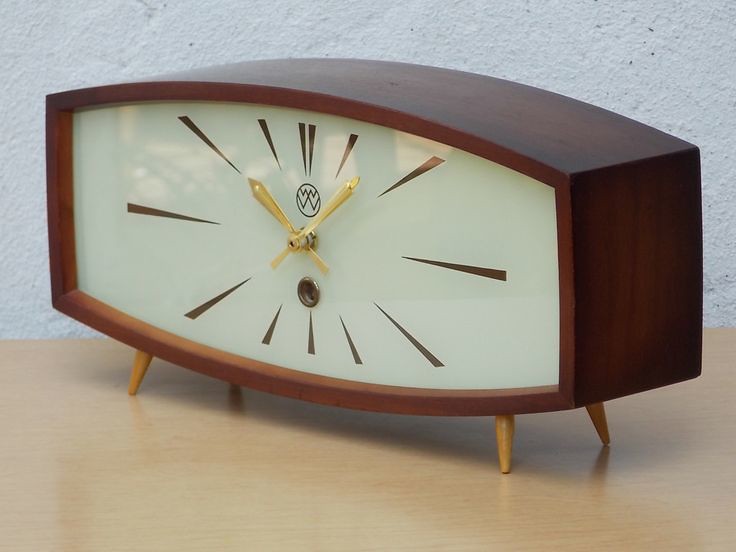A meticulously designed tabletop clock is elegantly positioned on a light wooden desk. The clock rests at a slight angle, facing to the left against a backdrop of a light blue, textured wall. This wall has a rustic finish, adding a touch of vintage charm to the scene. The clock itself features a unique, bubbled rectangle shape, with its top and bottom slightly curved and its width greater than its height. It boasts a pristine white face, covered with a glass casing that reflects light subtly. The clock's hands are crafted from gold, adding a hint of sophistication. Instead of numbers, minimalist brown lines denote the hours. Notably, there's a small winding hole, indicating that it might be wound manually. Encased in dark wood, the clock sits sturdily on four short legs, giving it a robust and balanced appearance.